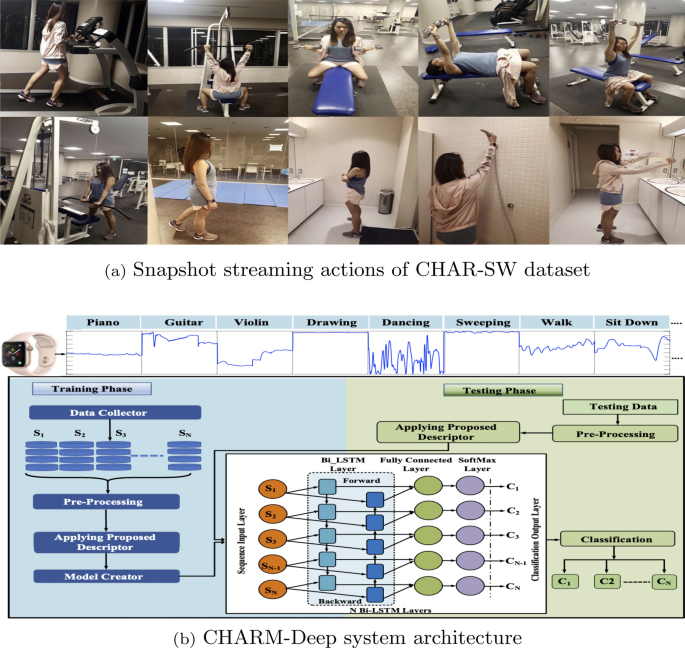The image features a photo collage comprised of approximately ten pictures showcasing a woman in various locations and activities, primarily centered around fitness. Each picture highlights her engaging in different exercises, including running on a treadmill, lifting weights, and performing curls and other gym routines on various equipment with distinct color details—white hoodie, blue undershirt, and white shorts. One image includes her washing up in a lavatory with white floors, countertops, and a silver trash can, and other shots depict her in the bathroom, including the shower with white walls and a silver showerhead.

Beneath the collage, the image contains a textual annotation reading "Snapshot streaming actions of char SW data set" in black text. Below this text is a schematic diagram presented against a background of alternating light blue and grey shades. The diagram broadly represents a data collection and diagnostics process and includes elements such as a training phase, data collector, and pre-processing descriptor model. Indicative icons and activities like piano, guitar, violin, drawing, dancing, sweeping, walking, and sitting down are highlighted, presumably to show heart rate or biometric measurements. The structured representation includes a variety of shapes and colors, including orange circles, blue and grey rectangles, and other graphical elements displaying the data set and its parameters on a predominantly blue and white background.